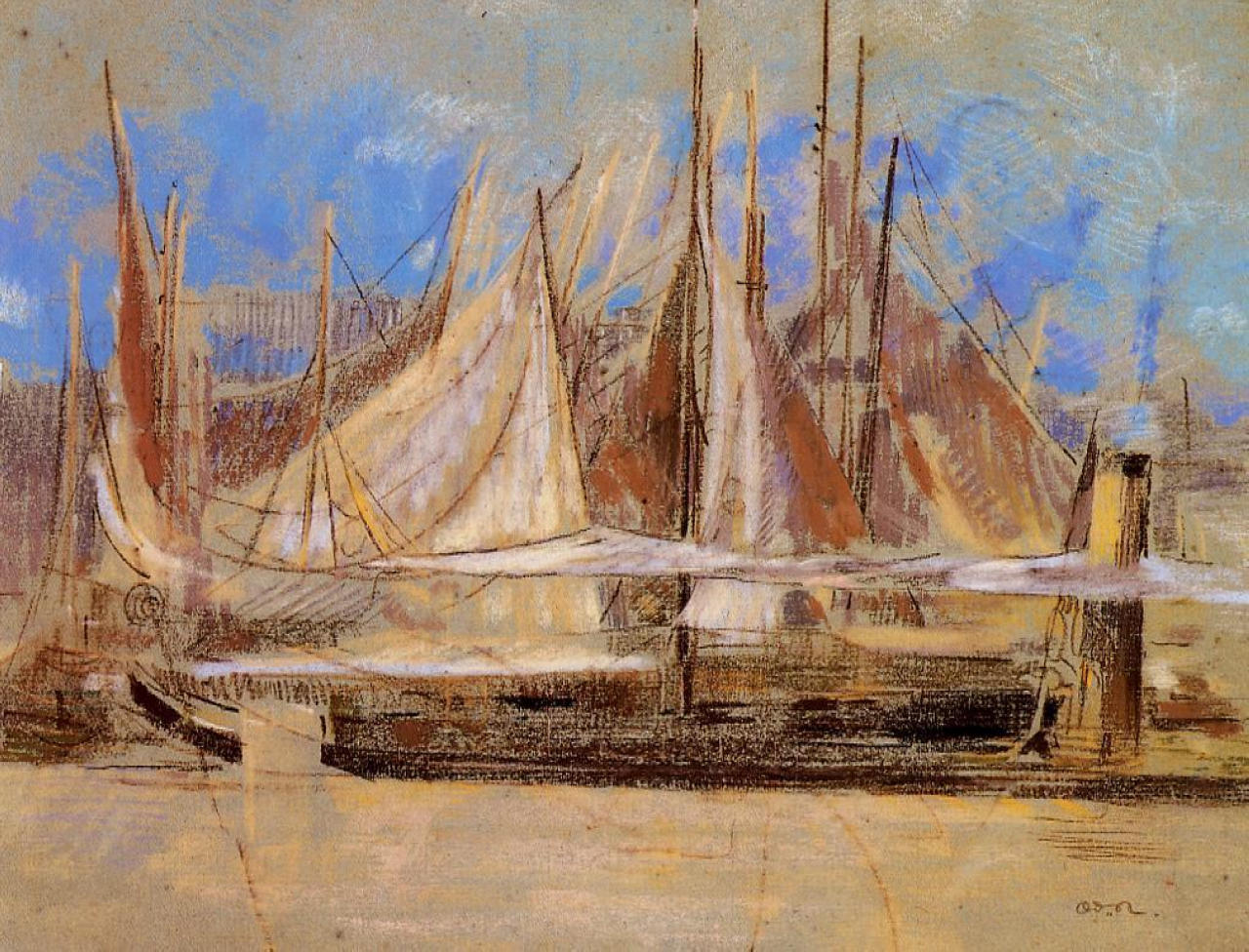This painting, titled "Yachts at Royan," features an outdoor setting depicted in a detailed and vibrant style. In the foreground, a brown plot of land sets the stage for a low, horizontal tent with a large pillar or column on the right side. Adjacent to this structure, a series of vertically positioned, triangular tents stand tall, painted in shades of brown and red. The background reveals a clear blue sky streaked with soft white clouds. In the central composition, what appears to be a large ship or several yachts, with dark brown bases and white, yellow, and brown overlapping sails, captures the viewer's attention. The sails, numbering about five or six, are lined up at what seems to be a pier or dock, shaded with streaks of brown. The elements of the painting are framed by a brownish hue on the left, possibly indicating a fence or posts, and a yellowish-brown color at the bottom, hinting at the wooden post or pillar mentioned earlier. The image carries the signature "O.D.R." in cursive at the bottom right corner, adding a personal touch to the artwork. Notably, there are no people present in this serene and meticulous scene, allowing the structures and natural elements to stand out prominently.